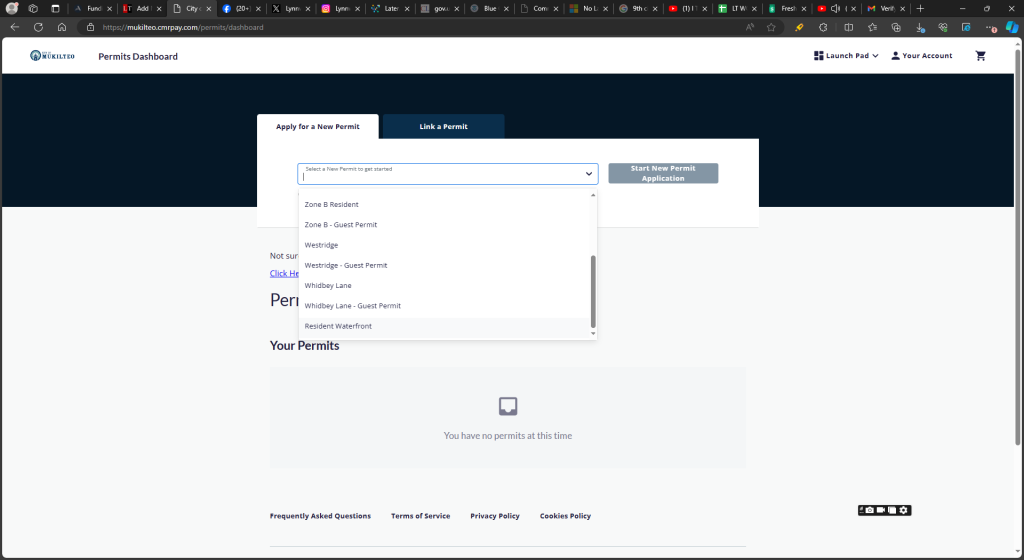At the top of this detailed web page, there's a narrow black bar stretching horizontally from left to right. This bar contains numerous tiny options and icons, though they are so small that they're difficult to read or identify. It also appears that the person has multiple tabs open, visible as small gray rectangles aligned parallel to the bar. Recognizable icons suggest that some of these tabs might include websites like Instagram and YouTube.

Beneath this black bar lies a search bar with unreadable input. Following this, there is a prominent blue rectangle spanning the width of the page. Centrally positioned over this blue area is a white square box, which contrasts against both the blue rectangle and the remaining white background of the page.

Within this layout, there are two tabs: the active one is white, while an unopened tab reads "Link a Permit". Below these tabs, there's a dropdown menu displaying a range of options, none of which are clearly legible. Text is slightly visible behind this menu, though it’s also unreadable.

Further down, the page displays a section titled "Your Permits," accompanied by a grayed-out icon resembling a square. This section states, "You have no permits at this time."